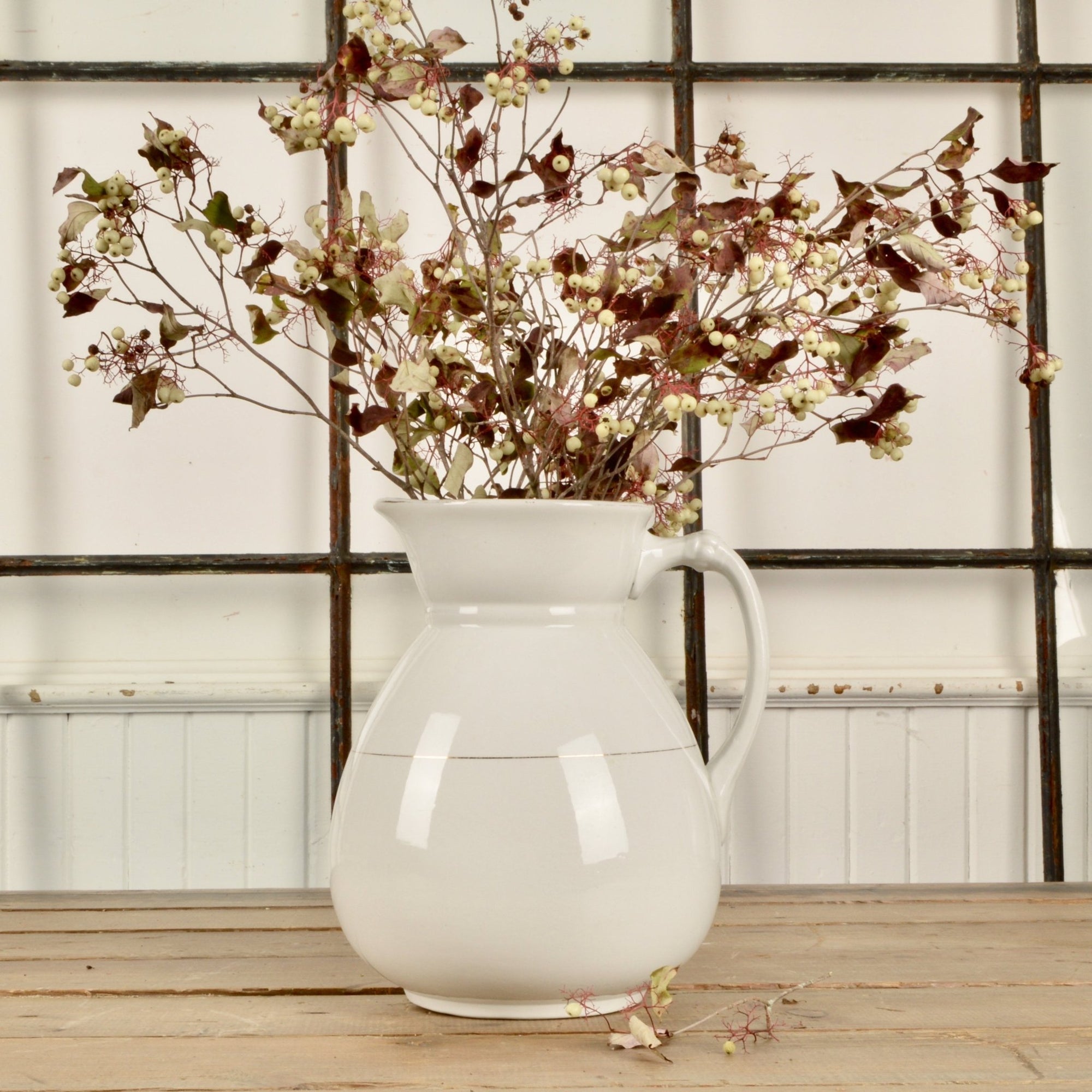This detailed photograph features a white pitcher, repurposed as a vase, resting on a light brown wooden table. The pitcher has a distinct section in the middle, held together by a wide strip of white tape, with a thin silver line running around it. The handle, positioned on the right, extends gracefully before reattaching near the base. Emerging from the top of this makeshift vase are spindly branches adorned with a variety of plants: long brown stems, amber-colored and reddish leaves, green shoots, and clusters of small white berries. Scattered beside the pitcher on the table are some fallen plant pieces. The background reveals a solid white wall with paneling near the bottom, and a set of rusted black metal bars arranged in squares, resembling a window frame with no glass. The muted tones and artistic arrangement suggest it was created for aesthetic purposes, conveying a sense of rustic charm and subtle elegance.